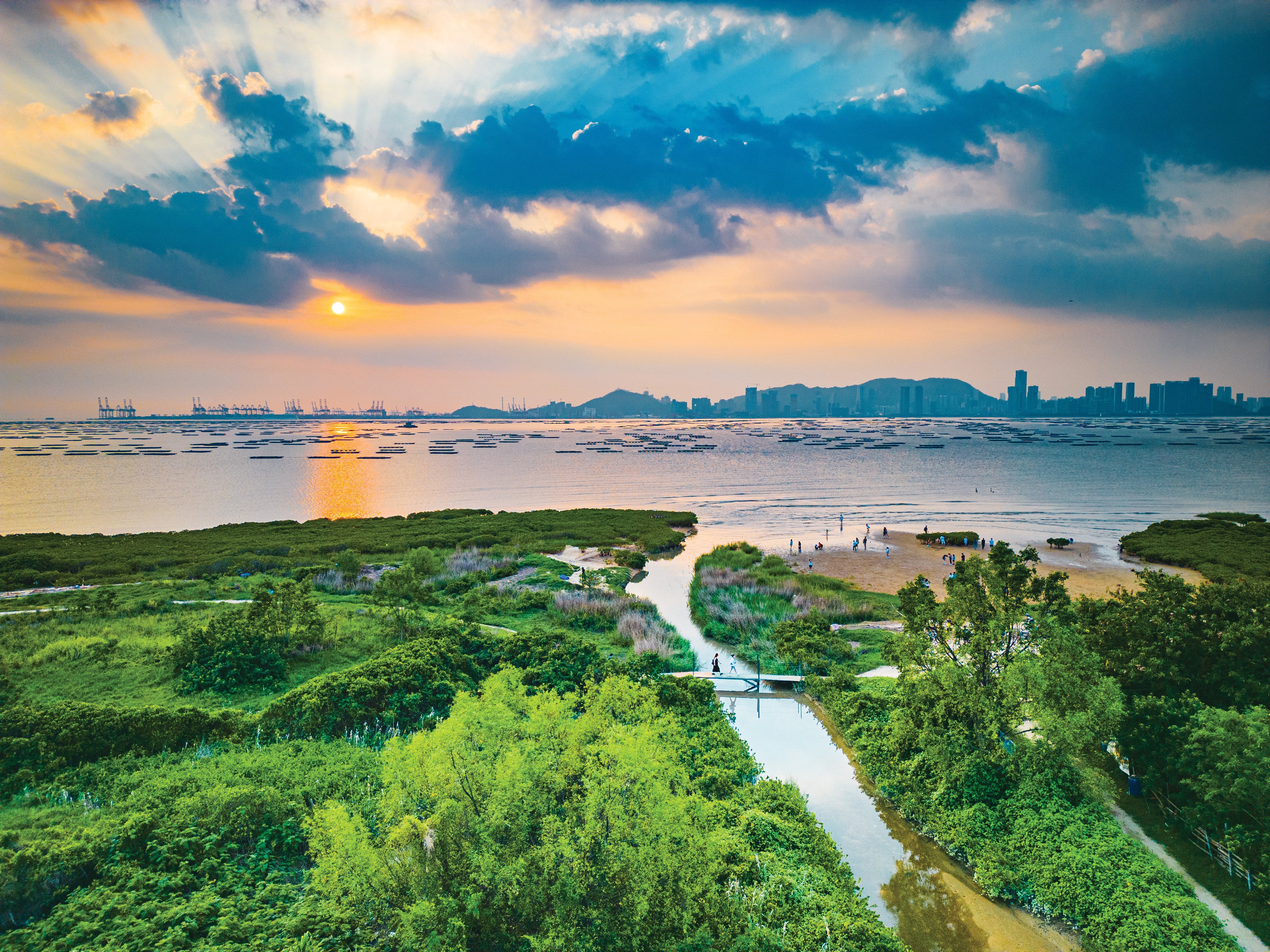This image, likely taken from a drone in landscape orientation, offers a striking bird's-eye view of a lush, green garden area descending into a large waterfront. At the bottom, the plush, vibrant grass and trees frame a small inlet of water that curves elegantly before merging into a vast body of water. Colorful bushes and flowers are nestled closer to the water on the left, while a sandy, beach-like area with a possible structure is visible on the right. A winding walking path begins from the right side, crosses a pedestrian bridge over a narrow canal, and stretches toward the sandy beach area. 

The middle of the image showcases an expansive bay filled with hundreds of small, flat boats anchored throughout the serene water. In the distance, a formidable city skyline, possibly Chicago, rises prominently, backed by large hills or mountains. Above this urban silhouette, the scene transitions to a dramatic sky displaying a mesmerizing sunset. The sun rests low on the left, casting rays through dark blue and grey clouds, with occasional patches of blue sky peeking through. The entire landscape, with its intricate details and vivid colors, resembles a breathtaking, almost painterly, natural and urban harmony.